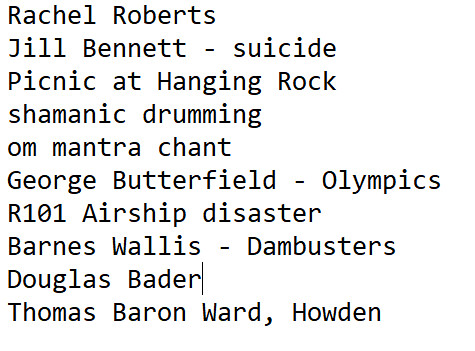The image features a plain white background with ten lines of text written in a bold, typewriter-style font. At the top is the name Rachel Roberts, followed by Jill Bennett - Suicide, Picnic at Hanging Rock, Shamanic Drumming, and OM Mantra Chant. Continuing the list, the names and details are George Butterfield - Olympics, R101 Airship Disaster, Barnes Wallace - Dam Busters, Douglas Bader, and the final entry is Thomas Barron Ward, Howden. This appears to be a set listing for a music concert, presenting the names of musicians alongside the titles of their performances or themes.